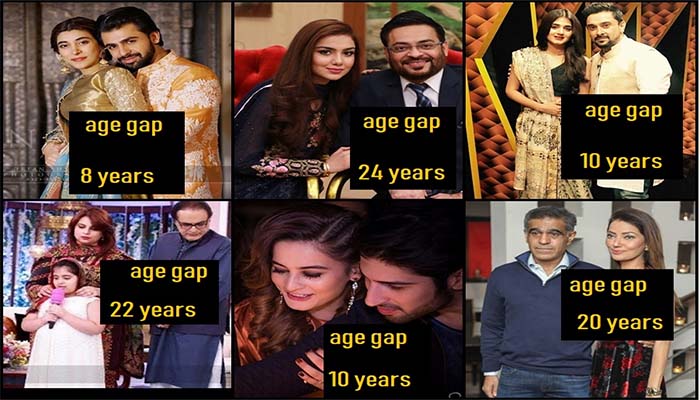The image is a rectangular collage consisting of six smaller photos, arranged in two rows of three. Each photo features a couple with a black square displaying the text "age gap" in yellow and indicating the number of years between partners. The couples seem to be of Indian or Middle Eastern descent, potentially wearing traditional attire.

- **Top Row:**
  - **Top Left:** A couple with an age gap of 8 years. The woman is dressed in a golden outfit, and the man is in an orange and white, shiny ensemble.
  - **Top Middle:** A couple with an age gap of 24 years. Both wear black outfits; the man has black hair, a black beard, and a mustache.
  - **Top Right:** A couple with an age gap of 10 years. The woman has long brown hair and wears a brown dress with an Indian style, while the man is in a tan vest.

- **Bottom Row:**
  - **Bottom Left:** A couple with an age gap of 22 years. The man and woman are positioned closely, with the woman standing behind a child.
  - **Bottom Middle:** A couple with an age gap of 10 years. They are closely positioned, mainly showing their heads.
  - **Bottom Right:** A couple with an age gap of 20 years. The man has his arm around the woman's waist, both appearing intimate.

All couples are depicted in close proximity, emphasizing the varied age gaps between them.